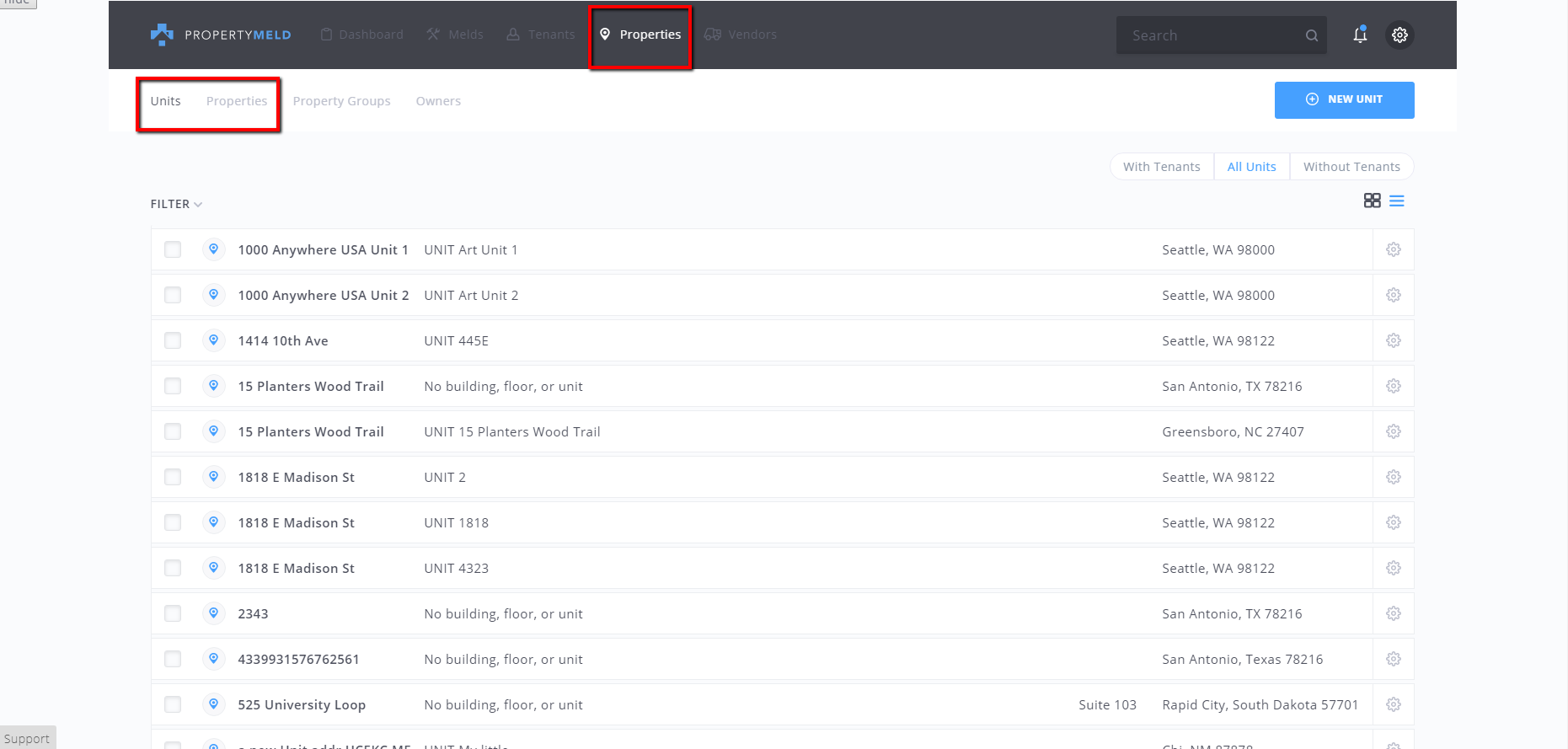This image is a screenshot of a web page from the "Property Meld" website. At the very top, the header menu is a very dark gray, almost black. On the right side of this header, the words "PROPERTY MELD" are written in white and blue capital letters respectively. To the left of these words is the company's logo, which consists of four squares arranged with two side-by-side, one at the top, and one at the bottom. There is a cutout in the logo that makes it resemble a house.

In the center of the page, a section is highlighted with a red line drawing a box around the word "Properties" which is written in white. To the left of "Properties," there is an icon in the shape of an inverted teardrop, indicating a location pin.

Beneath the header, on the left side, the words "Units" and "Properties" are present, with a red rectangle drawn around them to highlight these sections. The remaining menu options, "Property Groups" and "Owners," are listed to the right of the highlighted words.

In the upper right-hand corner, beneath the dark gray header, there is a rectangular button with the words "NEW UNIT" written in white.

On the left side of the page under a "Filters" header, there is a list of property addresses. The cities corresponding to these addresses are displayed on the right side. The cities listed at the top include Seattle, Washington (appearing three times), San Antonio, and Greensboro, North Carolina, among others.